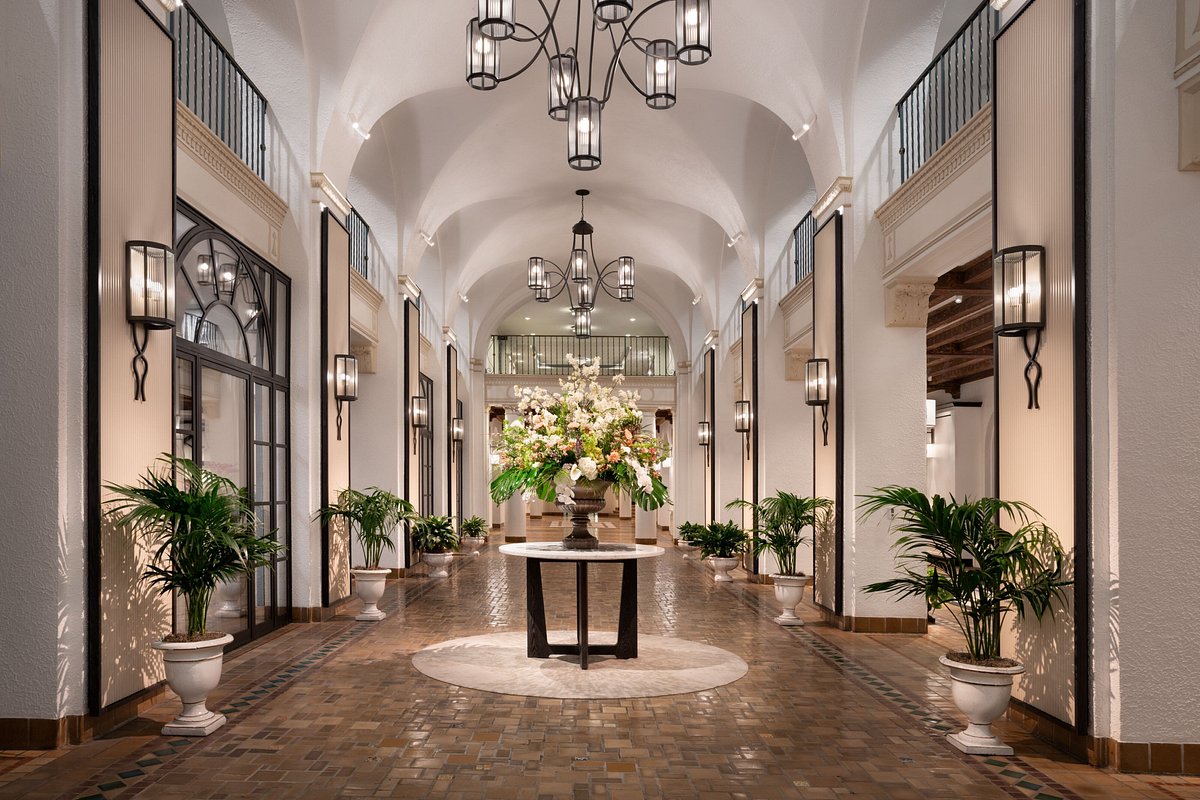This photograph captures a grand and ornate hallway or entranceway, likely within a large home, hotel, or convention center. The floor features a brown, small stone pattern with green diamond accents and brown edging. Flanking the hallway are large windows with potted ferns in white urns next to them. Ornate black and glass sconces adorn the walls beside the entrances on either side, and overhead, silver and glass chandeliers hang majestically.

At the center of the hallway lies a round table with a white top and brown legs, positioned on an off-white circular rug. A striking floral arrangement in shades of white and green serves as the table's centerpiece. Potted palms or ferns, placed in matching white urns, line the hallway, creating a symmetrical and inviting path.

The perspective of the photograph leads the eye towards a vanishing point, highlighting the depth and grandiosity of the space. The hallway extends to reveal different entrances on the left and right, each framed by additional potted plants and sconces. The upper level of the hallway features black wrought iron railings, adding an element of elegance and reinforcing the hall's two-story height. Overall, the ambiance is both luxurious and welcoming, perfectly blending natural elements with intricate design.